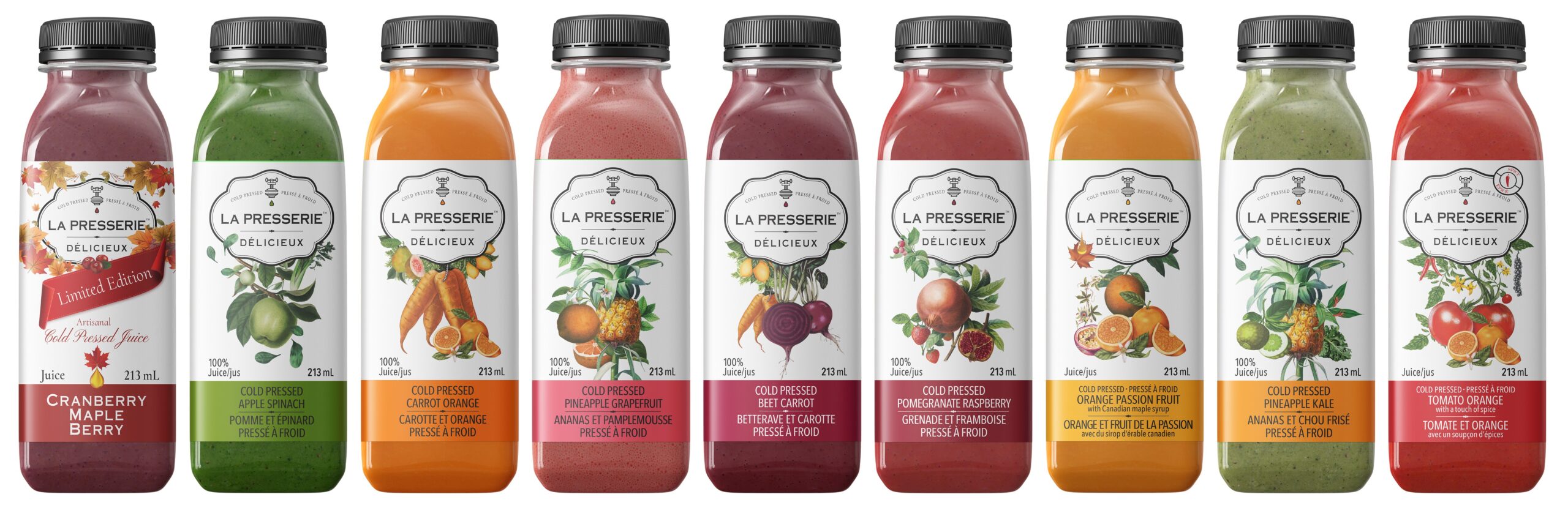The photograph displays nine identical bottles lined up against a white background. Each bottle is the same size and shape, featuring black tops and white labels bearing the "La Presserie" logo. They differ in color and content, representing various juice flavors. Starting from the left, the bottles are filled with the following juices: cranberry maple berry (dark red or violet), apple spinach (green), carrot (orange), pineapple grapefruit (light red), beet (another dark red), pomegranate raspberry (not-so-dark red), orange passion fruit (yellow-orange), pineapple kale (off-green), and tomato orange (ruby red). The labels also depict various fruits and vegetables corresponding to each flavor, making the vibrant array of juices visually appealing and suggestive of their diverse, delicious contents.